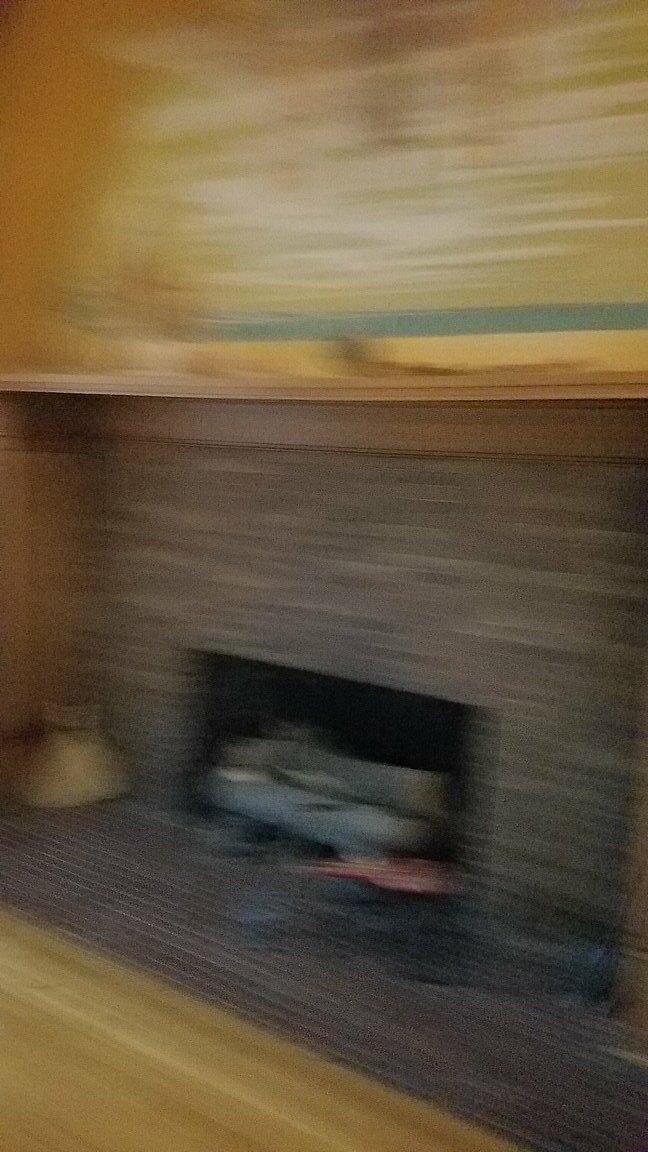This image is a very blurry, out-of-focus photograph depicting a cozy living room scene centered around a brick fireplace. You are viewing the fireplace from an angle, where it extends from the bottom right towards the bottom center of the left side of the image. The bricks of the fireplace appear to be dark, possibly reddish-brown to brown and tan, though the blur makes it hard to discern precise colors. Inside the fireplace, two logs are set vertically, with another red object visible beneath them, leaning against the brickwork. 

A wooden mantelpiece, in a warm golden, chocolatey brown hue, runs horizontally above the fireplace. Below the mantel, there is a smaller wooden ledge. Above the mantel hangs or is part of what seems to be more wood paneling, potentially adorned with a forest green stripe, although the swirling blur of the image makes it challenging to be certain. Near the fireplace on the left, there's a blurry shape that could be a stuffed animal, a cat, or some sort of pot. To the right side of the fireplace, there might be tools for tending to the fire. The floor in front of the fireplace is a light wood grain, matching the blonde wood paneling suggested above. The photo has the characteristic look of being taken with a shaky hand, resulting in its extremely blurry and motion-like quality.